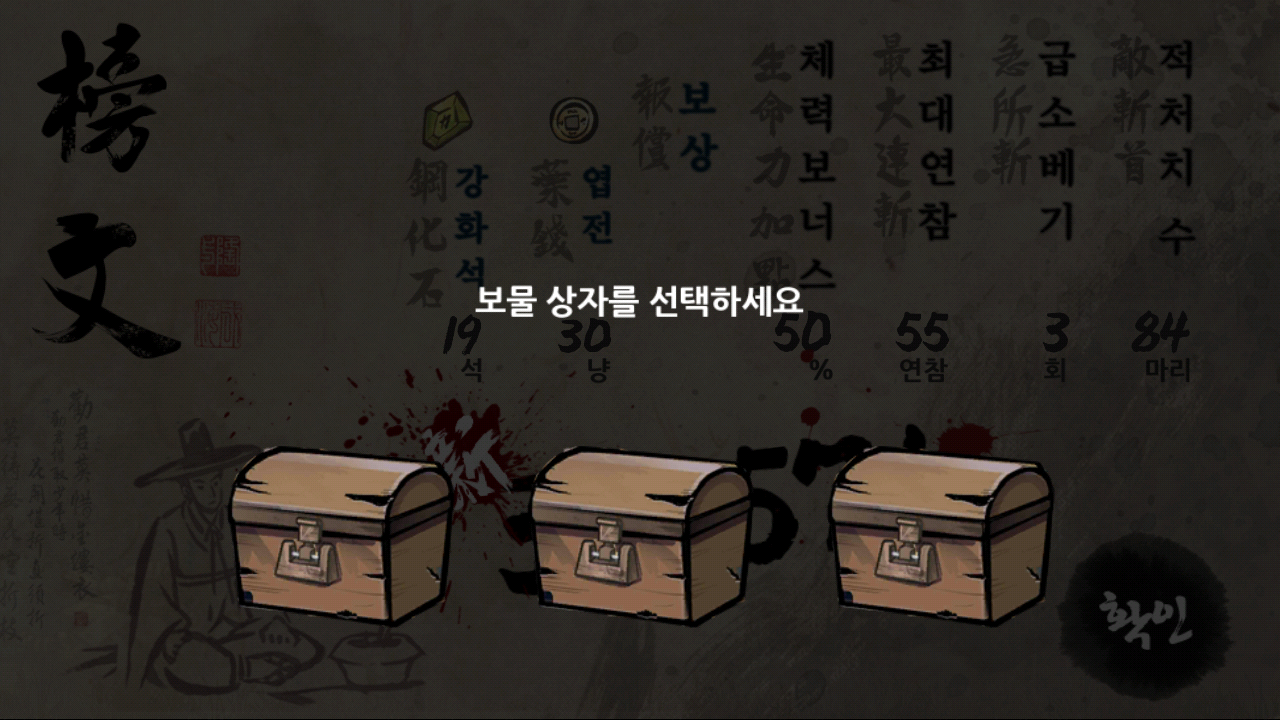The image is a detailed digital illustration resembling a screenshot from a video game, likely a treasure hunt adventure. The background is a deep, dark charcoal gray adorned with subtle silhouettes of Asian characters, suggesting a possible Japanese or Korean origin. Across the bottom of the image, three small, light brown wooden treasure chests are aligned horizontally. These chests, which feature latches and stress marks to add authenticity, hint at an interactive element typical of video games. In the center of the image, white text written in an Asian language, possibly Korean, stands out against the dark background. The background also contains faded numbers such as 19, 30, 50, 55, 3, and 84 among the subtle calligraphy, adding layers of intrigue to the scene.